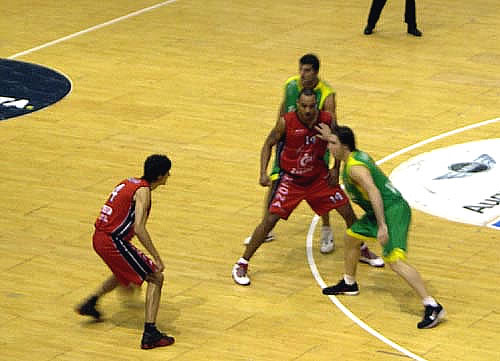This photo captures a dynamic moment in a professional basketball game on a standard wooden court, distinguished by visible logos and lines. In the center of the image, four players are intensely focused on the play. Two players clad in red, black, and white uniforms are positioned against two players in green and yellow uniforms. The red player's team predominantly features red in their attire, while the green player's team has black and white sneakers with complementary highlights.

The red team player in the bottom left, identified as number 4, appears to be dribbling the ball with his left hand. A shadow under his left knee hints at the ball's motion. He is wearing black sneakers with red accents. Directly in front of him, another red team player, numbered 14, is receiving defensive pressure from a dark-haired Caucasian player in green, who has his hand pressed firmly against number 14's chest. This player in green is in a ready stance, while his teammate is also focused on the play.

The court also features several visible logos, including "AU" encased within a blue bar with a yellow stripe on the right side, and a prominent black circle with a thin white stripe and a white "A" on the left side. A figure in black pants and black shoes, likely a referee, is partially visible in the background, enhancing the game's official atmosphere.